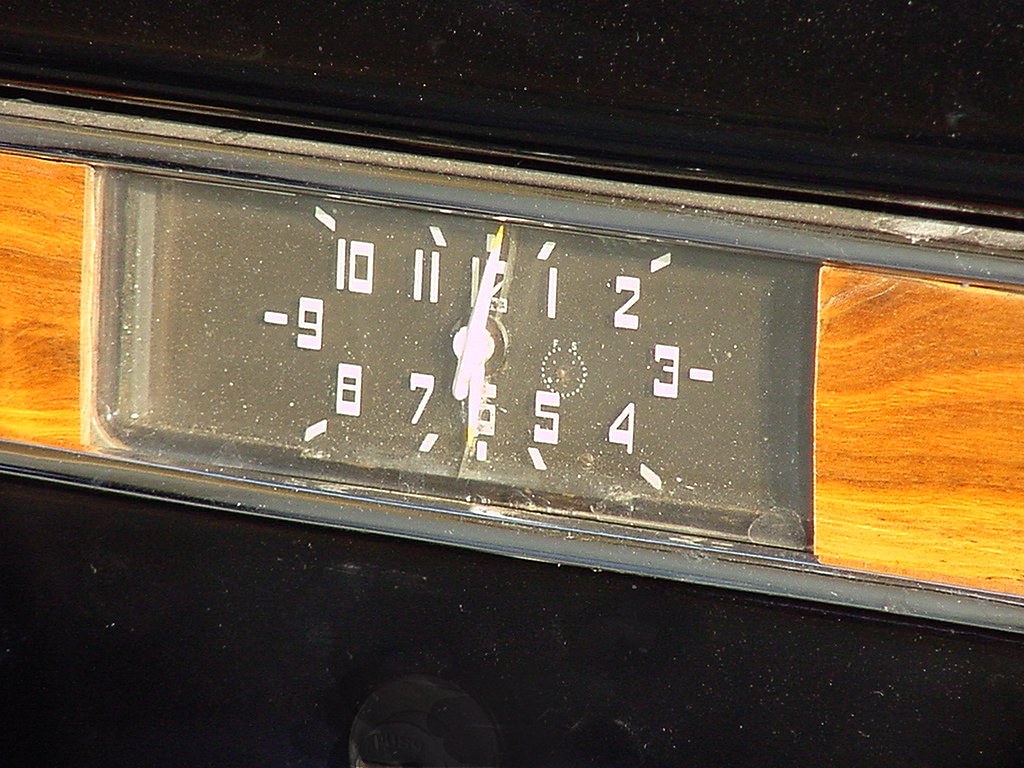The image features an antique-style clock with a distinctive design. The clock has a metal frame on both the upper and lower parts, giving it a vintage look. The sides of the clock are cropped out of the picture, which is taken at a slight angle, tilting to the right. This positioning makes the left side of the clock appear slightly elevated compared to the right. The frame around the clock face is made of a thin, metal-looking plastic, while the sides, which are visible, showcase a wooden texture. The clock's hands indicate the time as 6:01. The entire composition exudes a nostalgic charm with its mix of materials and skewed perspective.